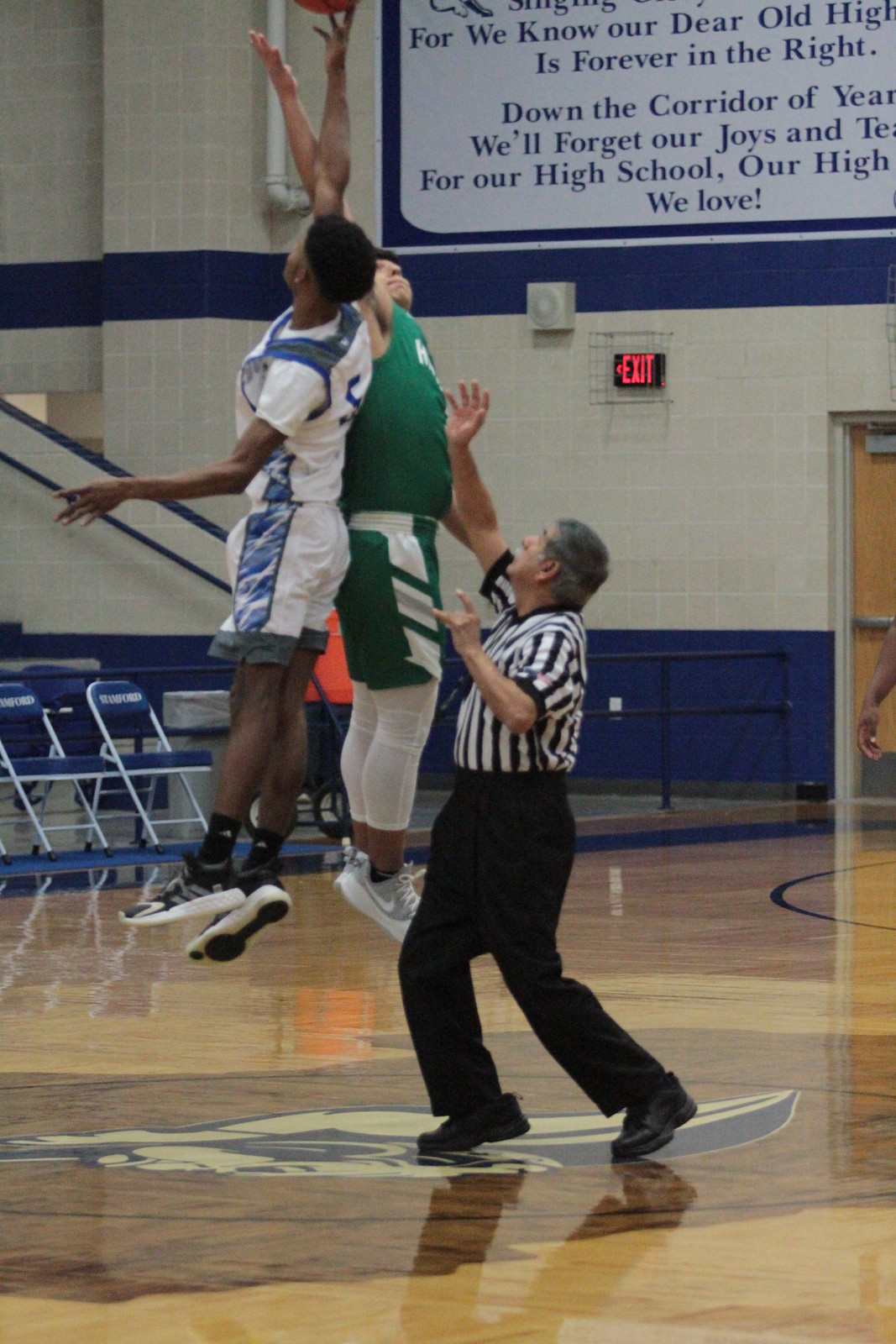This detailed color photograph captures an indoor scene of a basketball practice game taking place in a school gymnasium. The focal point of the image is two young boys, one African-American wearing a white and blue uniform with black shoes and socks, and the other possibly Asian or Caucasian or Latino, dressed in a green uniform with white accents, white shoes, and what seems to be yoga pants under his shorts. Both boys are airborne, stretching out their arms as they vie for a basketball, which is partially visible at the top left of the image.

Positioned centrally is a middle-aged referee with gray hair, clad in the customary black and white striped shirt, black pants, and black shoes. His right arm is extended as he monitors the action closely. In the background, the gymnasium’s polished hardwood floor gleams under the lights. The walls and decor feature the school’s blue and white colors, including blue and white folding chairs and a large, partially visible mural. A red LED exit sign and a large wooden door also adorn the background. The overall scene presents a vivid moment within a typical school sporting environment, accentuating the dynamics of a jump ball under the attentive eye of the referee.